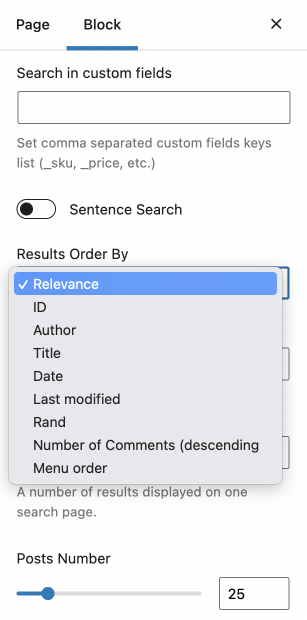This image appears to be a screenshot from a software application or website interface designed for content management, particularly for blocking certain pages or websites. The interface features two main tabs at the top, labeled 'Page' and 'Block,' with the 'Block' tab currently selected. 

In the upper-right corner, there's an 'X' button likely used for closing the window. Below this, there's a search bar labeled 'Search in custom fields,' accompanied by a text box with grey placeholder text that reads, "Set comma-separated custom field keys list (e.g., _SKU, _price, etc.)."

Beneath the search bar, there's a toggle switch labeled 'Sentence search,' which is currently in the off position. Following this is a section titled 'Results ordered by,' featuring a list of sorting options. The first option, 'Relevance,' is selected and highlighted in blue, while the other options include 'ID,' 'Author,' 'Title,' 'Date,' 'Last Modified,' 'RAND,' 'Number of Comments Descending,' and 'Menu Order.'

Further down, greyed-out text indicates an option for 'Number of results displayed on one page,' followed by a numerical value and a slider set to 25. Partially obscured by the dropdown list are additional text boxes, the functions of which remain unclear.